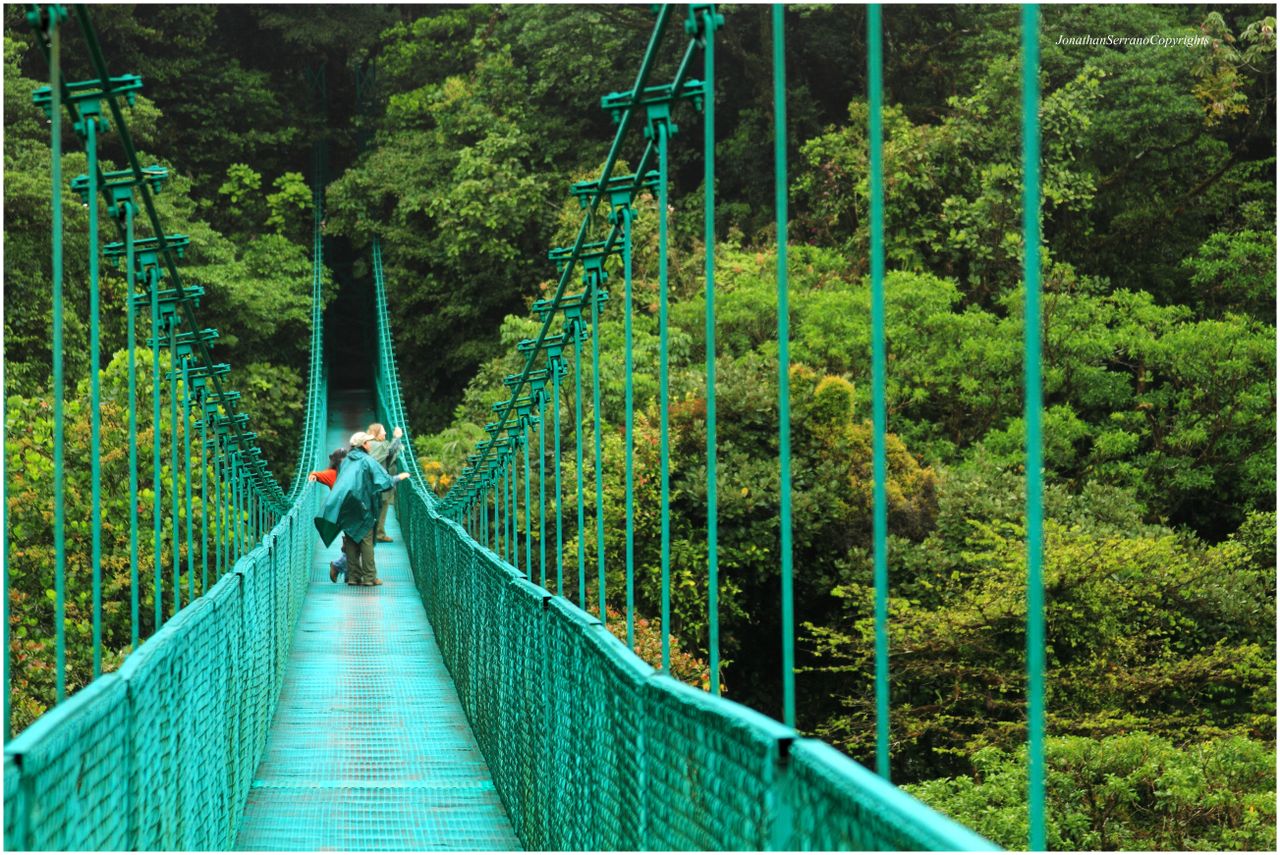This photograph captures an old-fashioned suspension bridge, designed for pedestrians and painted a now weathered and scuffed teal hue. The bridge spans from the bottom left corner of the image and stretches diagonally into the dense forest that engulfs the background. It's presumed to cross over a river or valley, though only the lush green canopy is visible. The bridge has wire railings and fencing that matches its light green-blue color, adding to its aged aesthetic. Three figures walk away from the camera on the far edge of the bridge: a woman in a large teal blue poncho resembling the bridge’s original color, and two children whose faces are not visible. They seem to be central to the image’s composition, standing at the part where the suspension cables dip down before rising again. The dense forest behind them is a mixture of light green and yellow hues, suggesting a vibrant and sunlit day. The scene is topped off with small white text at the top right corner, reading "Jonathan Sereno Copyrights," discreetly marking the photo.